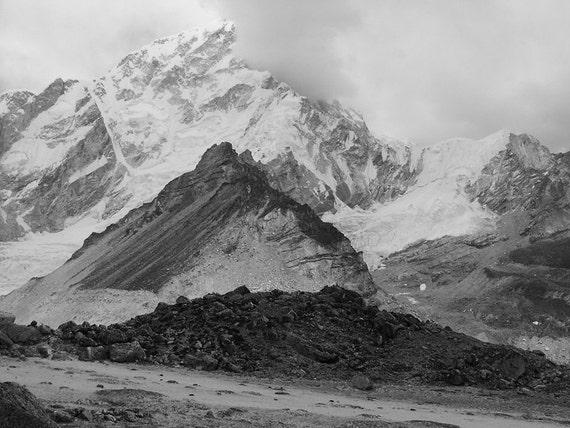This black-and-white photograph presents an outdoor mountainous scene that captures a natural, untouched landscape. The composition reveals a clear delineation between foreground, middle ground, and background, bringing depth to the image. In the foreground, there is a stretch of dark dirt and rock, stripped of any snow, possibly indicating a road that blends into the rugged terrain. Moving to the middle ground, the mountains start to show traces of snow, their surfaces becoming increasingly chiseled and jagged. In the background, towering peaks dominate the landscape, their summits blanketed in snow, contributing to the impression of a high-altitude environment. The largest of these peaks occupies the upper left quadrant of the frame, heavily laden with snow. Overhead, the gray, murky sky is filled with dense, floating clouds, suggesting an overcast day. While the scene evokes the glaciers found in places like Alaska, there are no specific markers to confirm the location. The stark contrast between the snow-covered mountains and the dark, rocky foreground hints at a seasonal transition, possibly early winter or late spring. All vegetation is absent, reinforcing the raw and rugged beauty of this mountainous expanse.